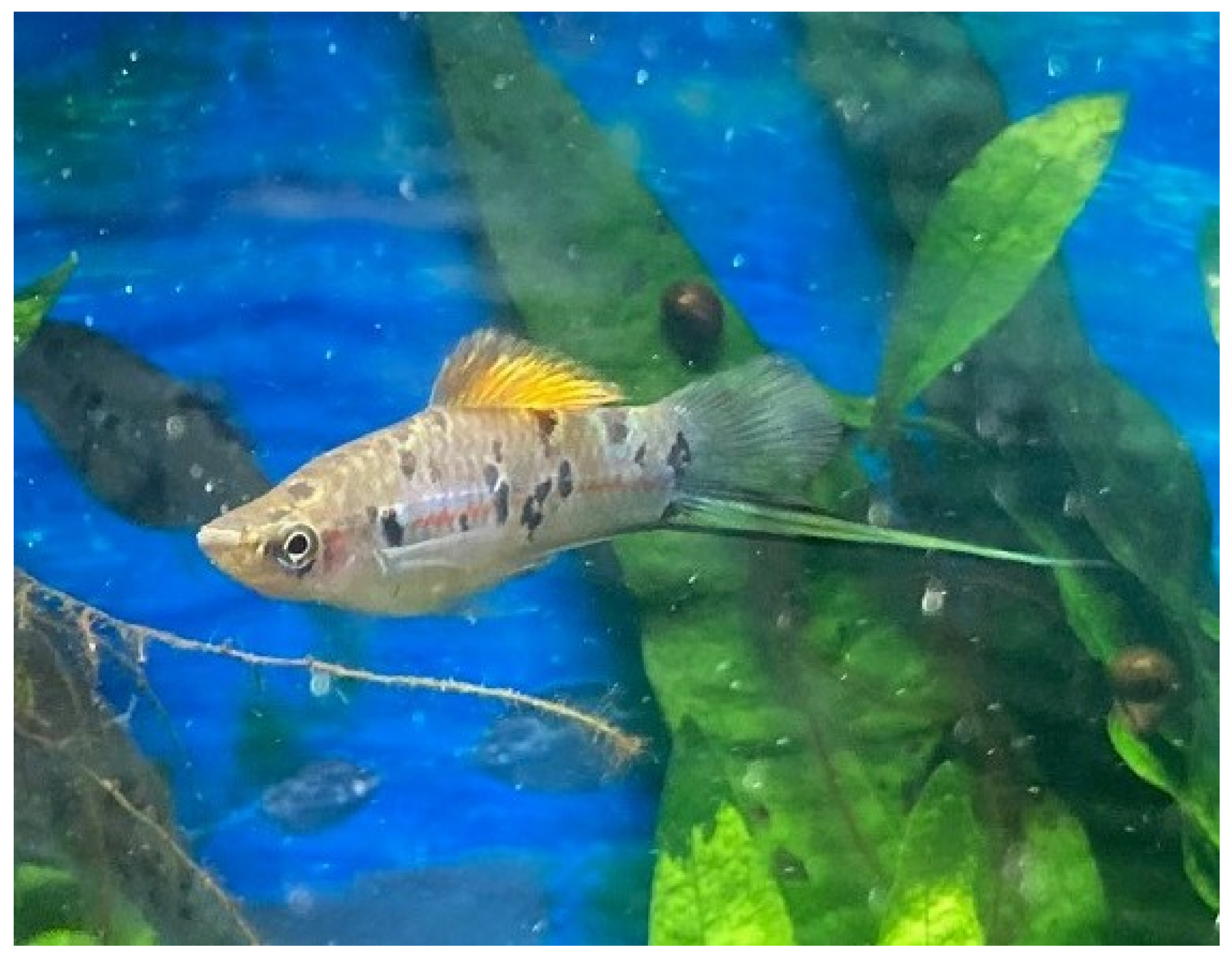The photograph is a detailed, full-color image, likely taken underwater, with a square aspect ratio. Dominating the center is a small tropical fish showcased in profile as it swims leftwards. The fish has an angular face with a pointed mouth and one visible eye of green-gold hue with a slight red tinge around it. Its body appears a mix of light tan, brown, and gray with distinct black spots scattered across its scales. The standout feature is its top fin, which is bright yellow with gray edging, complemented by a translucent back fin. Another notable fin, resembling a long, thin green leaf with a black border, extends beyond its tail. Surrounding the fish is a backdrop of blue water interspersed with green leafy seaweed and some plant roots visible directly below, adding to the aquatic ambiance of this vibrant underwater scene.